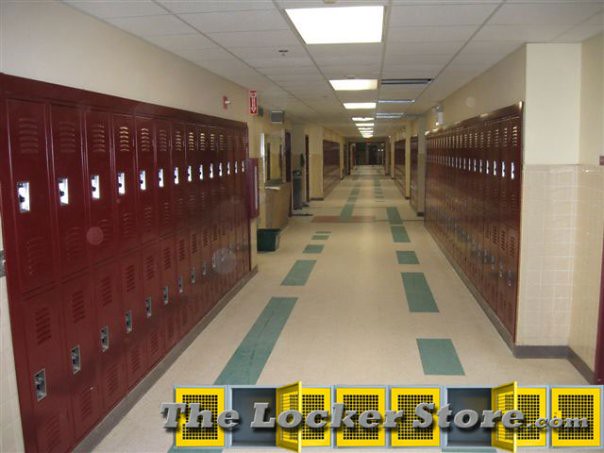This image depicts a typical hallway in an American middle or high school. The hallway features a beige floor adorned with green rectangular patterns that run its length. Flanking the corridor are rows of lockers: red lockers on the left and right sides with an extensive series stretching into the background, where a blurred exit sign is visible. Each locker has a visible combination lock area and vent lines at the top. The corridor's walls above the lockers are painted beige, complementing the drop tile ceiling fitted with long fluorescent lights that illuminate the space evenly. In the lower right corner of the image, there is a logo or a web address, "thelockerstore.com," written in light gray. This text, along with the open and closed yellow lockers behind, gives the image the appearance of an advertisement. Overall, the scene epitomizes the typical, somewhat monotonous ambiance of a school hallway, devoid of windows and any ornamental features.